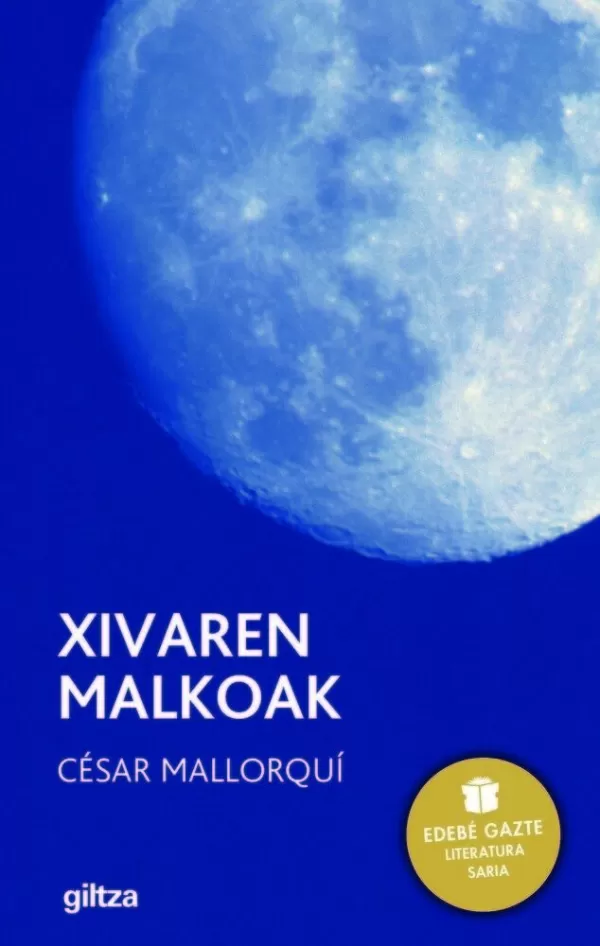This detailed cover image consists of a deep royal blue background, featuring an image of a celestial body occupying the upper right half of the cover. The celestial body, likely the moon due to visible craters on its surface, is depicted prominently. The title of the book, "Ixvarin Malkoic," and the author's name, "Cesar Mallorqui," are both inscribed in white text on the cover. Below the author's name, the word "Giltza" appears. In the lower right corner, a yellow circular icon displays a book and includes the phrase "Edebi Gatsi Literaturia Saria."